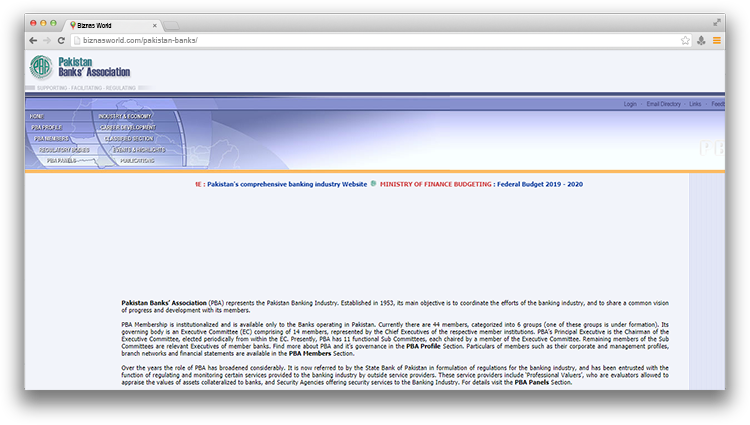This image depicts a web page that appears to be a part of a banking and industry website, specifically linked to the Pakistan Bank Association. At the very top, the page features a prominent logo of the Pakistan Bank Association. Below this logo is a bluish toolbar with a background that includes an intricate pattern, possibly featuring a globe.

The toolbar contains a menu with ten different options, albeit with blurred text. The readable menu items include "Home" and other categories which are not fully legible. Underneath the toolbar, there is a header stating "Pakistan's Comprehensive Bank and Industry Website."

Following this header, there is another link related to "Ministry of Finance Budgeting, Federal Budget 2019-2020." The central portion of the page consists of an open space that separates the header and toolbar from the main content.

The main content area seems to split the page into two halves, presenting paragraphs that elaborate on Pakistan's banking industry and the website. Certain words within these paragraphs are highlighted in bold, while the majority of the text remains in regular print.

At the very top of the browser window, the tab indicates that this web page might be accessed through an older version of Internet Explorer, characterized by the specific design elements typical of that browser.

Overall, the image captures an older styled web page from the Pakistan Bank Association, featuring a structured layout with a focus on banking and financial information, set against a somewhat dated browser interface.